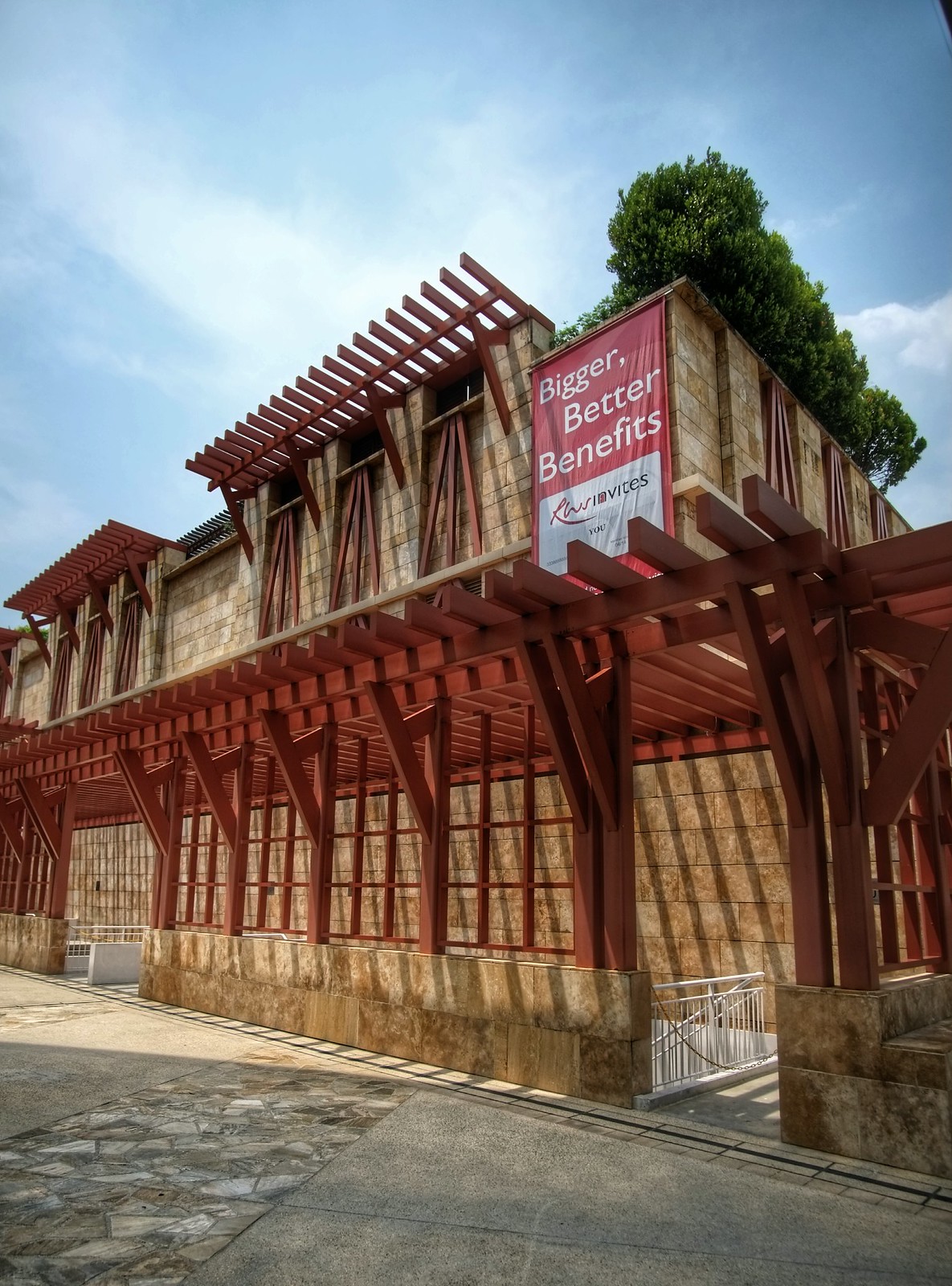The image portrays a two-story commercial building shot in portrait orientation from across the street. The structure, characterized by its light brown stone bricks and horizontal wooden planks, incorporates numerous dark reddish-brown stained wood beams. Indicating possible construction or a minimalist architectural design, the building’s façade lacks visible windows and has wooden structural elements revealing some plywood, suggesting it might still be under construction.

A distinctive feature is a large banner hanging from the top right corner of the building, vertically aligned along the height of the second floor. The banner is red on top with the white text "Bigger, Better Benefits" and a white bottom section displaying an illegible logo.

The street in front consists of a mix of concrete and cobblestone, enhancing the rustic aesthetic. A small, roped-off stairway descends from the building's entrance. Atop the structure, green trees peek out, suggesting an upper outdoor area. The sky above is clear with blue hues and scattered white clouds, adding to the serene, untouched ambiance, further emphasized by the complete absence of people in the scene. This photographic representation reflects a contemporary, unfinished building within a serene outdoor setting.